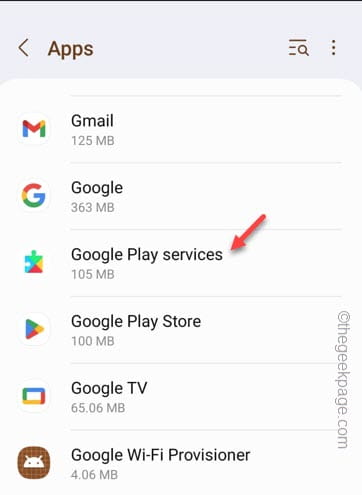The image displays a screenshot of an apps menu on an Android cell phone. The reason it is identified as an Android device is due to the prominence of Google app listings, which are characteristic of Android rather than Apple devices. At the top of the screen, the "Apps" setting is selected on the menu bar. To the right side, there is a clickable search bar and the familiar three vertical dots icon, which typically opens an extended menu with more options.

Below the "Apps" section, a list of installed applications is displayed, along with the amount of storage each app is occupying:

- **Gmail:** 125 MB
- **Google (Search):** 363 MB
- **Google Play Services:** 105 MB (highlighted with a red arrow)
- **Google Play Store:** 100 MB
- **Google TV:** 65.06 MB
- **Google Wi-Fi Provisioner:** 4.06 MB

Adjacent to the list of apps, on the right side of the screen, there is faint, gray text displaying “@ TheGeekPage.com”.